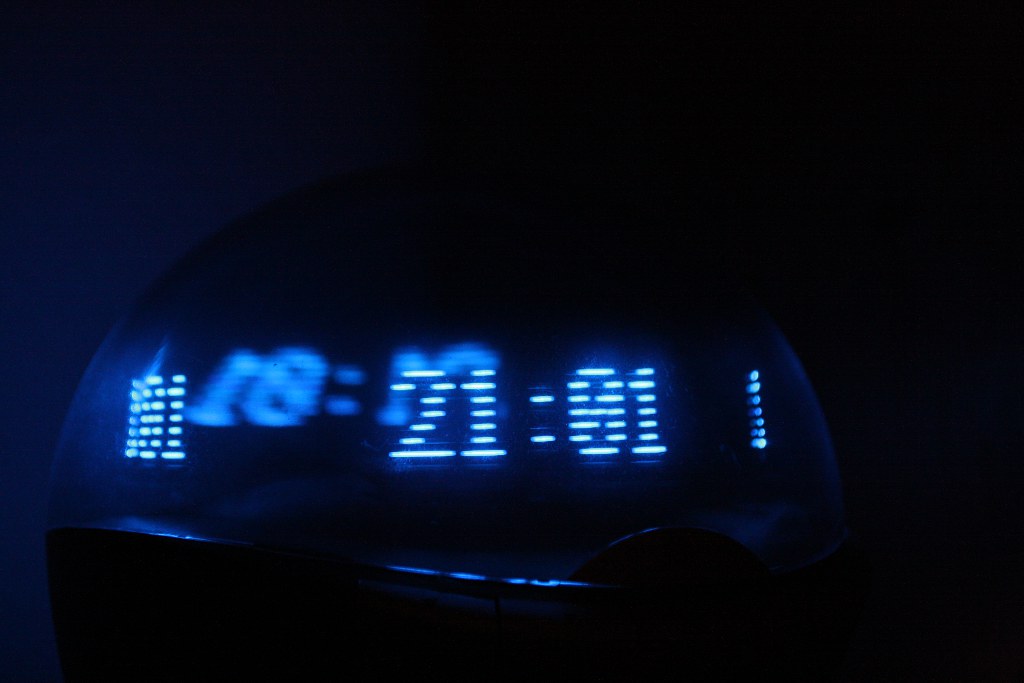The photograph is a color image likely taken inside a dimly lit room, possibly at night. It focuses on a unique circular alarm clock situated against a wall. The bottom half of the clock is shrouded in near-black darkness, while the top portion appears like a glass globe illuminated in dark blue. The central part of the clock glows with striking blue digital numerals and vertical lines, displaying a time of 21:01, meaning 9:01 PM. Below this, another set of numbers reads 01-21-01, which might represent a date. The illuminated globe-like face of the clock also reflects a faint light pattern toward the upper left, showing an ambiguous time of 18:12. Additionally, there are small vertical dots forming a square on the left side and a vertical line on the right, all radiating a similar bluish hue. The reflection on the clock's surface subtly reveals two windows with sunlight peeking through the blinds, adding a faint touch of external light to the dark, atmospheric setting.